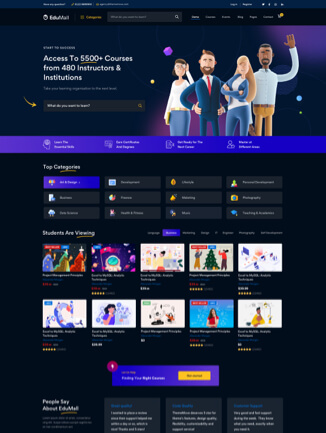At the top of the image, a banner showcases four distinct claymation figures. From left to right: 

1. A woman with brown hair, dressed in a pencil skirt.
2. A man sporting a blue suit, red tie, and brown beard.
3. Another woman, who has her arms crossed, wearing a denim jacket over a white undershirt with jeans.
4. Finally, a man with dark brown hair, khaki pants, a brown leather belt, and a blue button-up shirt.

To the left of these characters, white text reads, "Access to 5500+ courses from 480 instructors and institutions." A curvy yellow underline emphasizes the "5500+," and there's small, undecipherable white text at the bottom of this section.

Below the banner, a search bar is prominently displayed. A yellowish-orange curved arrow, reminiscent of the Amazon arrow, points towards the search bar. An orange magnifying glass icon is located on the right side of the bar.

Beneath the search bar, there's a gradient strip that transitions from purple on the left to dark royal blue on the right. Below this strip, white text on the left reads "Top Categories," underlined by the same yellowish-orange curve. Twelve rectangular options follow, each with a dark gray background except for the first one, which features the same purple-to-blue gradient as the strip above. The specific text on these options is too small to discern.